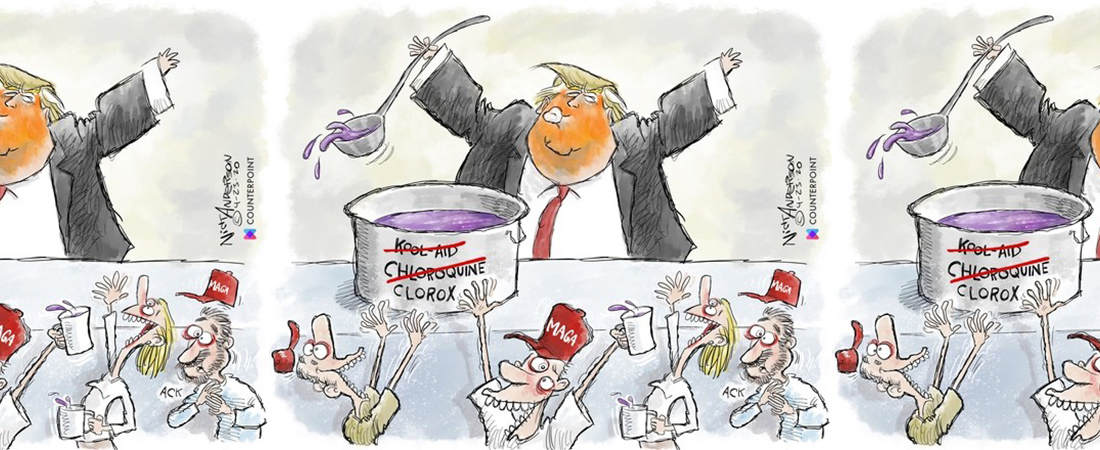The image is a political cartoon displayed three times in a row, with the central image fully visible and the side images partially cut off, all set against a white background. The cartoon depicts Donald Trump, characterized by his orange face, blonde hair, white shirt, red tie, and black suit jacket. Trump is standing behind a white table with both arms raised, making a kissy face. In his left hand (right from his perspective), he holds a ladle dripping purple liquid. In front of him, on the table, is a pot containing purple liquid labeled "Kool-Aid," "Chloroquine," and "Clorox," with the first two terms crossed out, leaving only "Clorox." Surrounding the table, a crowd of people wearing red MAGA hats are eagerly holding up cups to receive the liquid, looking euphorically crazed—all except for one man on the right who appears to be coughing and in distress, and another man on the left rushing forward to get a cup, as he doesn't have one.